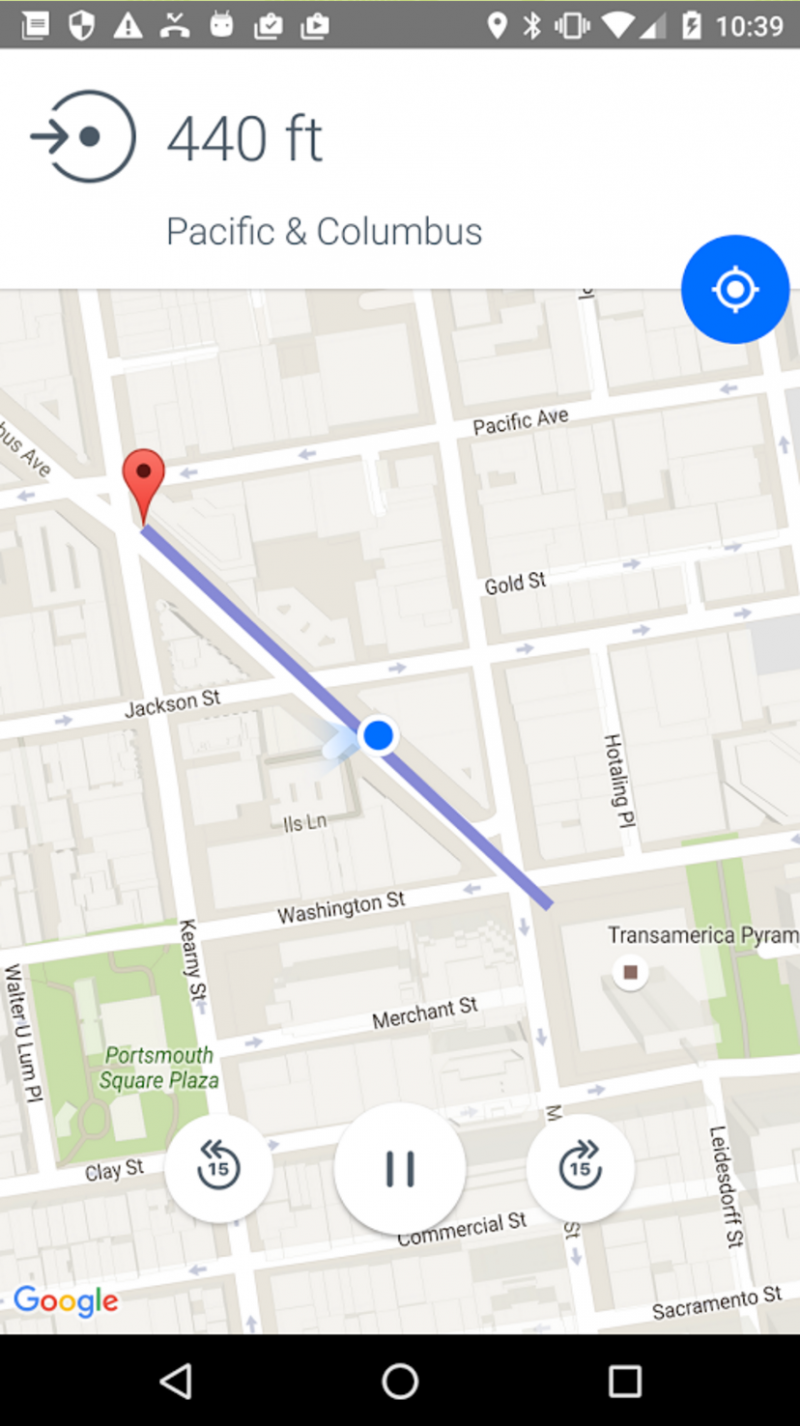A vertical screenshot taken on a smartphone showcases a detailed street map. At the top of the image, a gray status bar displays several icons, including the time, which is 10:39. The main section of the screenshot features a street map with a diagonal purple navigation line connecting two points. A red marker signifies the starting point, and a blue circle is displayed at the center of the map. 

Above the map, a white banner contains a directional arrow and a circular icon with a gray dot, indicating a distance of 440 feet between Pacific and Columbus. The map includes labeled streets such as Jackson Street, Pacific Ave, Gold Street, Washington Street, Portsmouth Square Plaza, Kearney Street, Merchant Street, Sacramento Street, and Commercial Street. 

At the bottom of the map, three white circles with icons overlay the image. In the lower left-hand corner, 'Google' is written in blue, red, yellow, and green letters. Below this, a black strip houses three additional icons, completing the interface of the screenshot.